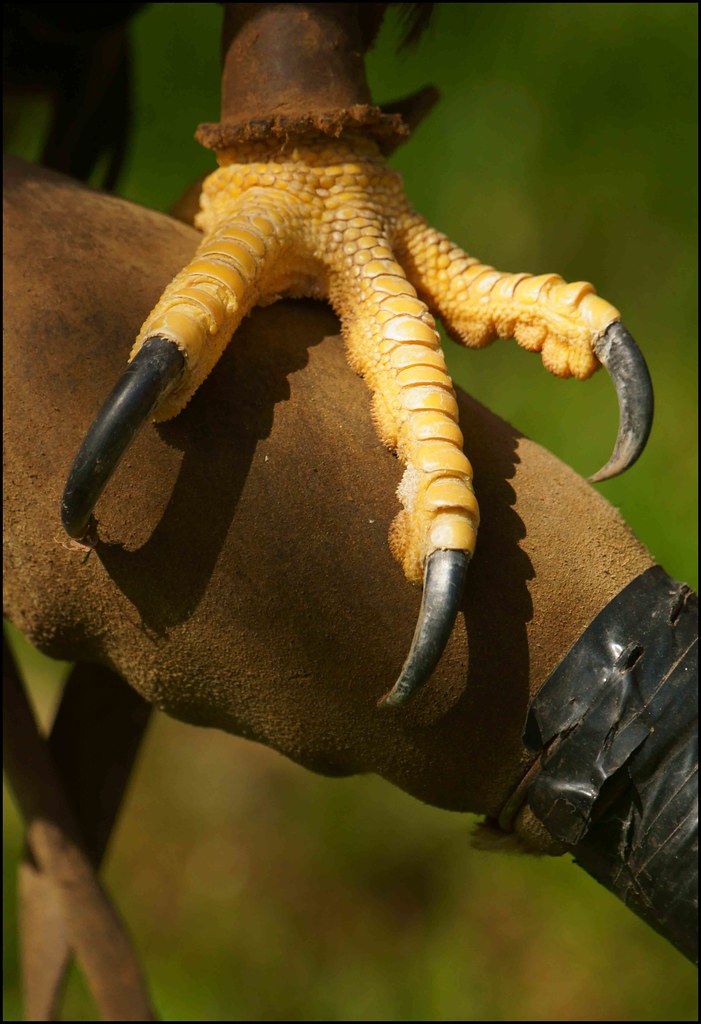The image features the talon of a large raptor, likely an eagle, firmly gripping its handler's leather-covered arm. The bird's three massive, black claws are prominently displayed, contrasting sharply with its golden, scaly toes. The talon is positioned on a brown leather falconry glove secured to the handler's arm with black duct tape. The glove effectively protects the handler from the bird's powerful grip. The background is a defocused green, suggesting the scene is set in a grassy or wooded area, though the exact details are blurred.